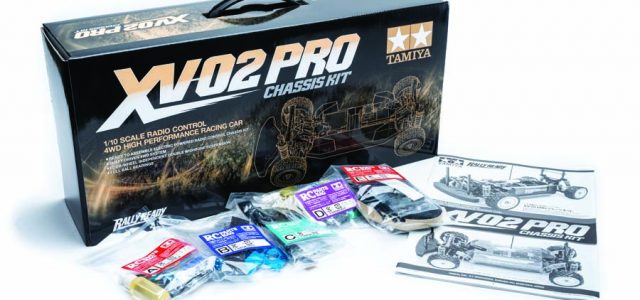This image features a boxed XV-02 Pro Chassis Kit by Tamiya, showcased against a white background. The black box prominently displays white and orange lettering, including the Tamiya logo, which features two stars in a tan and orange square. At the top of the box, it indicates "1/10th Scale Radio Control 4WD High Performance Racing Car" and features an image of the car. The center of the top has a cardboard handle. Below the box, five clear plastic packages are lined up, each containing different kit components with colored stickers: yellow (with a red sticker), blue, green, purple, and the last package again with a red sticker. To the right, a black-and-white manual labeled "XV-02 Pro Chassis Kit" is visible. The shadows of the box and packages cast onto the white background add depth to the image, providing a clear view of the contents meant for assembling the RC car.